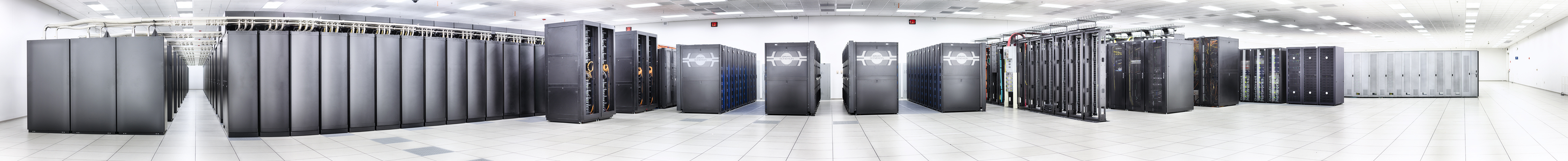The image shows a long and narrow room filled with rows of gray cabinets arranged in an orderly manner, suggesting an industrial or perhaps computer storage setting. The space is brightly illuminated by fluorescent lights, making the white tiled floor and ceiling stand out in the sterile atmosphere. The cabinets, which vary slightly in height and width, are primarily used for storage and feature gold handles in the middle of some units. Some cabinets are open, revealing shelves and orange coiled cords inside. The room, which could be part of a store or a large computer server facility, has paths between the rows for easy access to the cabinets. In the background, a couple of exit signs are visible, enhancing the sense of isolation in this vast, cold, and sterile environment.